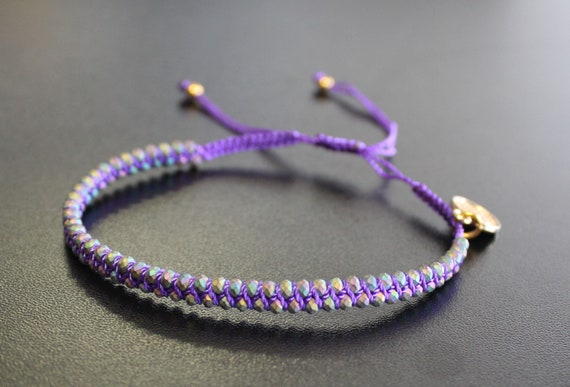This color photograph features a close-up view of a simple yet intricate friendship bracelet, laying on a dark gray backdrop. The bracelet is composed of purple thread and showcases a braided or knotted design. It is circular in shape and adorned with small, pastel-colored knots in yellow, green, red, and blue that intersperse the purple thread. A prominent gold circular charm dangles from the right side of the bracelet, attached by a loop. The bracelet culminates in two tassels, each tipped with a gold bead, though these beads appear blurred in the background. There are no other designs apart from the knots and gold embellishments, approximately 40 in total, that give the bracelet its distinctive textured appearance.